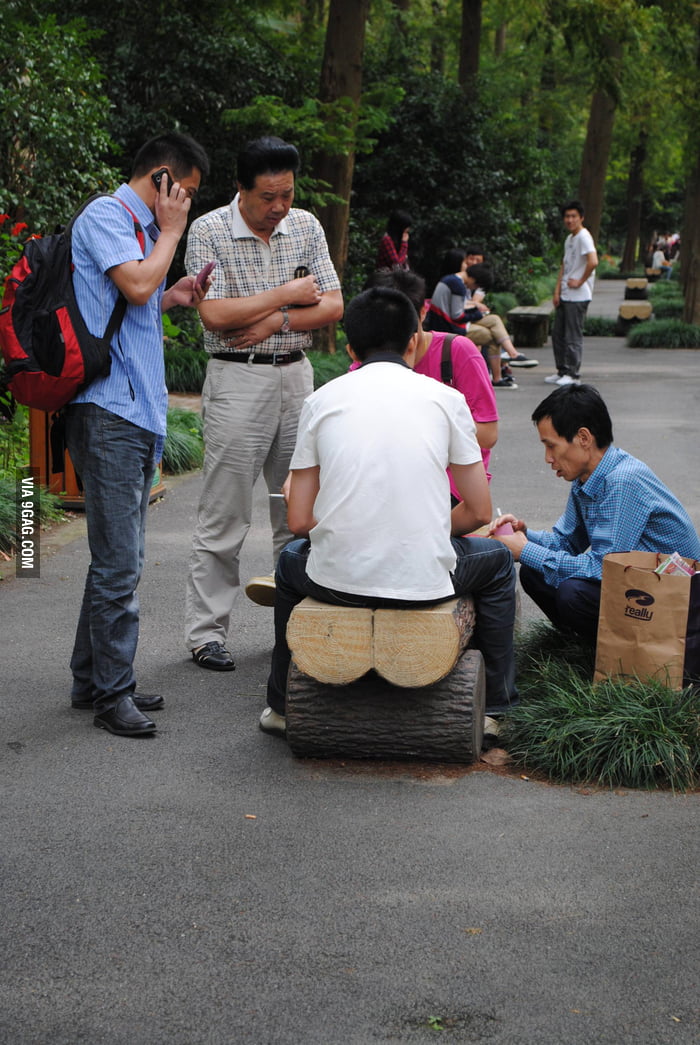The image features a group of Asian men congregated around a central asphalt walkway in a public park, surrounded by lush, dense greenery. The scene is vibrant, with colors such as gray, brown, green, blue, pink, and red prominently featured. At the forefront, two men are seated on a makeshift bench constructed from two logs stacked on top of a larger log, humorously resembling human buttocks. One man seated on this bench wears a white t-shirt, jeans, and beige shoes, while his companion, positioned opposite him, dons a pink t-shirt and a backpack. Flanking them are three other men; the leftmost is using his cell phone, and next to him, another man observes what the two on the bench are handling, though the exact object remains unclear. To the right of the bench, a man crouches with a paper bag branded "Really." The image, tagged via9gag.com, captures the casual gathering amidst nature, blending the mundane with a touch of humor.